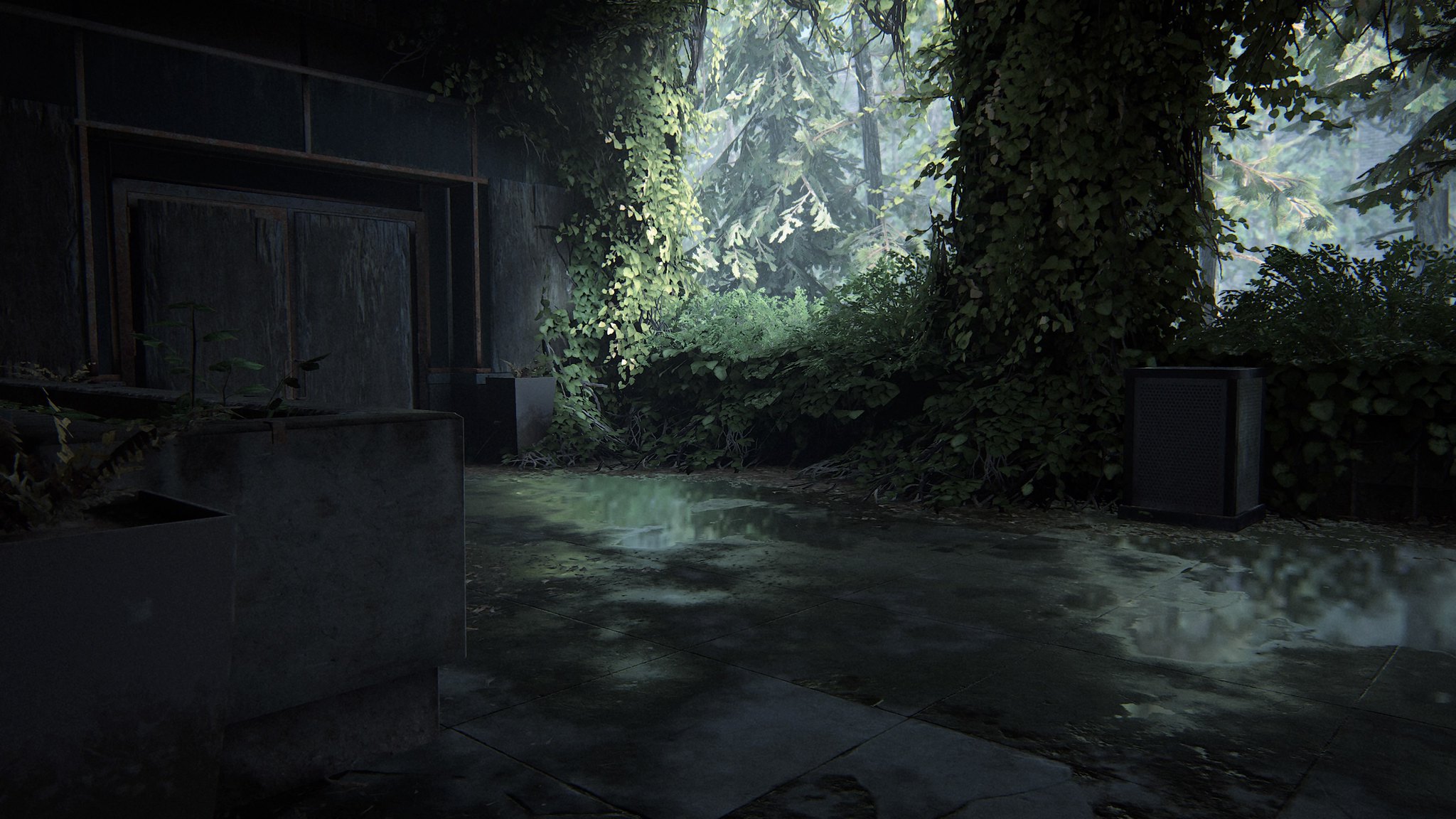This image appears to be an artistic illustration of a dark, enigmatic scene featuring a stone house with a garage door. The house is constructed from large blocks of brick, while a weathered stone wall topped with a planter and wild weeds adds to the rustic atmosphere. A driveway, seemingly wet from recent rain, adds a liquid-like shimmer to the scene, with wisps of fog or smoke rising subtly from its surface. A cement garbage pail with black trim stands near a towering tree, which is heavily adorned with ivy. The house itself is also entwined with ivy, enhancing its mysterious charm. The only light in the scene comes from scattered sunlight filtering through the tree canopy, casting a faint glow on an evergreen tree and some tree trunks in the background. The light accentuates the puddles on the driveway, contributing to the smoky, ethereal effect.